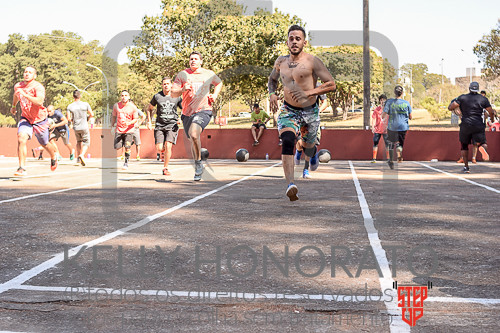The image captures a group of men running on a sunny day, on a concrete surface marked with white lines, likely in a park setting surrounded by green trees and a low fence in the background. Prominent in the foreground is a shirtless man wearing multicolored shorts and a knee brace, energetically striding with one leg on the ground and the other mid-air. Next to him, a man in an orange shirt and black shorts mirrors his vigorous pace. Further back, men in red tank tops and other colorful attire are also sprinting, their determined expressions highlighted by the mix of sunlight and shadows cast across the scene. A gray and red logo watermark, reading "Kelly Honorato" alongside a "step up" logo featuring a set of weights, is visible on the photo, adding a professional touch to this dynamic depiction of communal exertion.